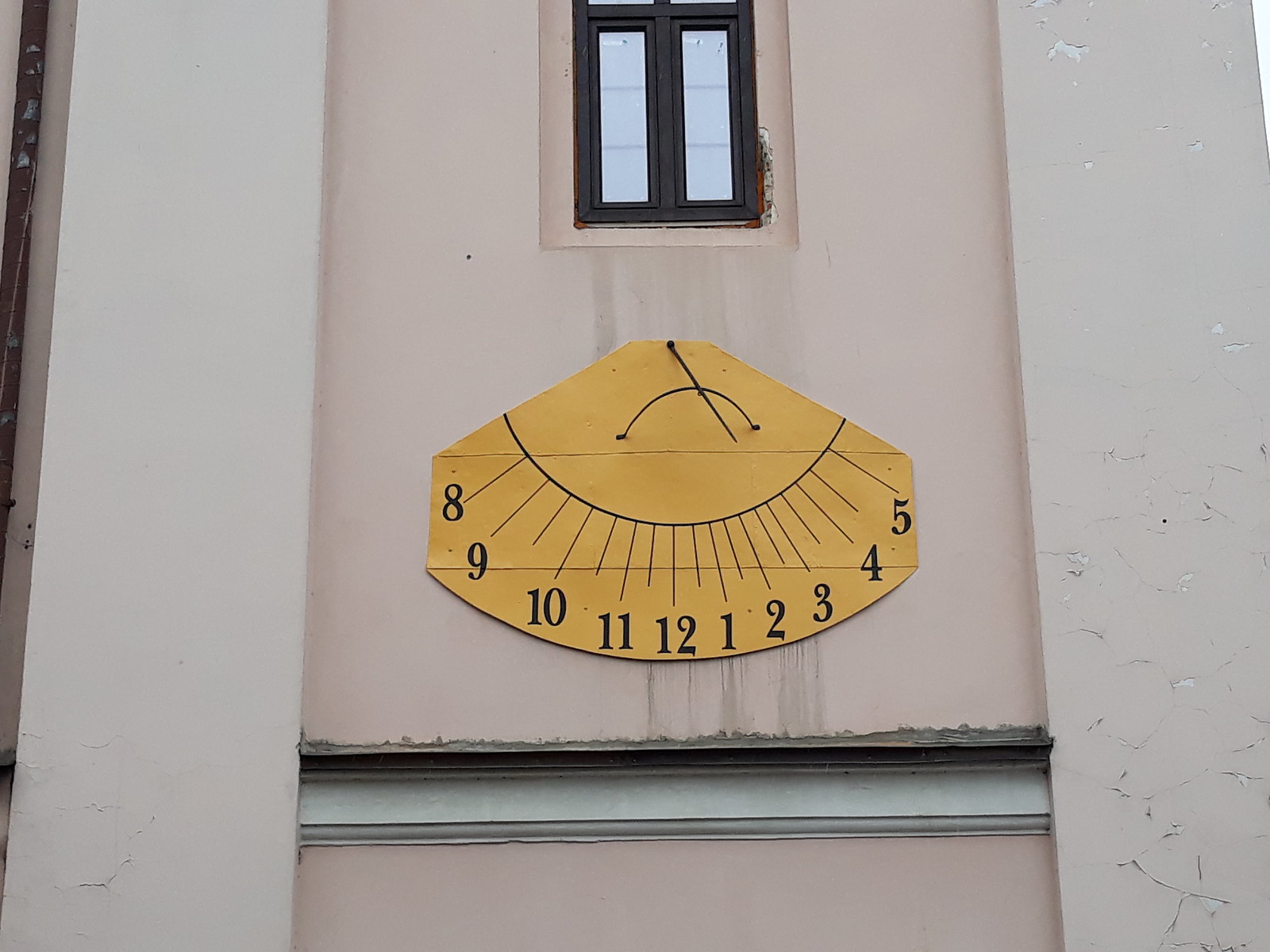The image showcases an outdoor wall adorned with a distinctly framed window at the top center. The window is framed with dark or black-painted wood, providing a stark contrast to the lighter elements surrounding it. On either side of the wall, two cream-colored columns stand, displaying signs of age and wear with visible cracking paint.

Beneath the window, the wall features a light pink hue. Dominating this section is a large, manila-yellow sheet of paper, shaped like the bottom half of a sun with radiating lines. Each line is numerically labeled, starting from the left with the number 8, and sequentially proceeding to 9, 10, 11, and 12 at the bottom center. The numbers then continue in an upward semi-circle from 1 through 5. The entire composition evokes a sense of time or a sundial-like structure, blending both color and form against the weathered facade.